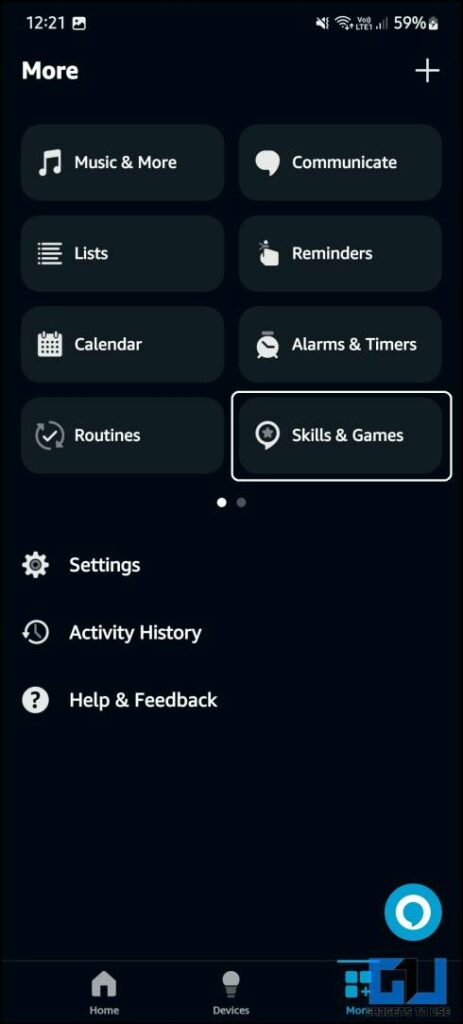This is a detailed graphical representation of a smartphone screenshot with a predominantly black background and white text. At the top, displayed on the left side, is the Instagram app icon, while on the right, the status bar reveals it is 12:21. The status indicators show a muted sound, a strong Wi-Fi signal, LTE connectivity, and a battery level at 59% alongside a battery icon.

In bold white text at the top of the screen, the word "More" is prominently displayed. Adjacent to it on the right side is a plus sign icon. The screen is divided into sections, each represented by dark gray rectangles. These sections include: "Music and more," "Communicate," "Lists and reminders," "Calendar and alarms," "Routines," and "Skills and games." The "Skills and games" option is highlighted with a light gray rectangle, indicating its selection. 

Beneath these sections are two dots, signaling the ability to toggle to the next set of options. Further down are additional functionalities: "Settings," accompanied by a settings icon, "Activity history," with a clock icon, and "Help and feedback," marked by a question mark icon.

At the bottom of the screen, navigation options are displayed in blue indicating selectable options for "Home," "Devices," and "More." The bottom right corner features a circular blue icon with a white circle inside it, housing a blue speech bubble that contains the stylized letters "G" and a mirrored "L" logo, both in blue.